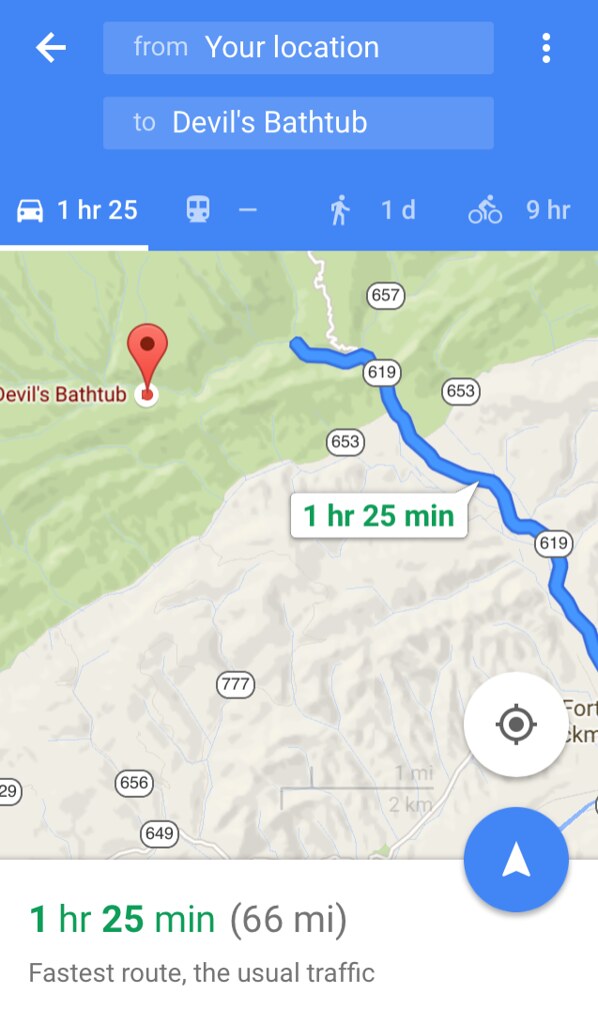In this detailed screenshot from a phone's navigation app, the top portion of the image features a blue banner displaying a car icon with the travel time listed as "1 hour 25 minutes," alongside a walking icon stating "1 day," and a bicycle icon indicating "9 hours." Below this banner lies a map, the upper half of which is green and the lower half off-white. Prominently marked in red on the green area is the destination, "Devil's Bathtub." A blue line traces the designated route from a starting point (indicated by a green arrow) through the off-white section. Various road numbers such as 619, 653, and 657 are visible along this path. Additionally, "1 hour 25 minutes" is reiterated next to the route. At the bottom of the image, further details include "1 hour 25 minutes," "66 miles," "fastest route," and "usual traffic."